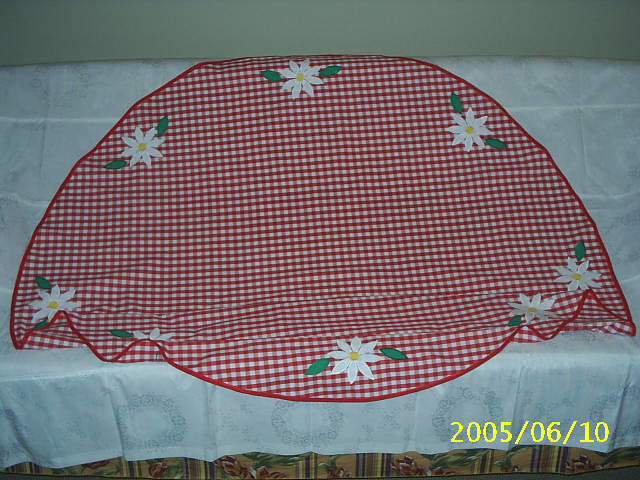The image captures a meticulously set table against a light gray wall. The table features a bottom layer with a wrinkly white tablecloth adorned with small round flowers arranged in a wreath-like design. Over this, there's a prominently placed tablecloth of an oval or umbrella-like shape, exhibiting a vibrant red and white checkered pattern. The border of this upper cloth is lined with white flowers featuring yellow centers and green leaves. At the very bottom of the image, part of another sheet peeks through, which is brown with green floral designs. Additionally, the date “2005-06-10” is clearly visible in yellow letters in the bottom right corner, marking June 10, 2005.